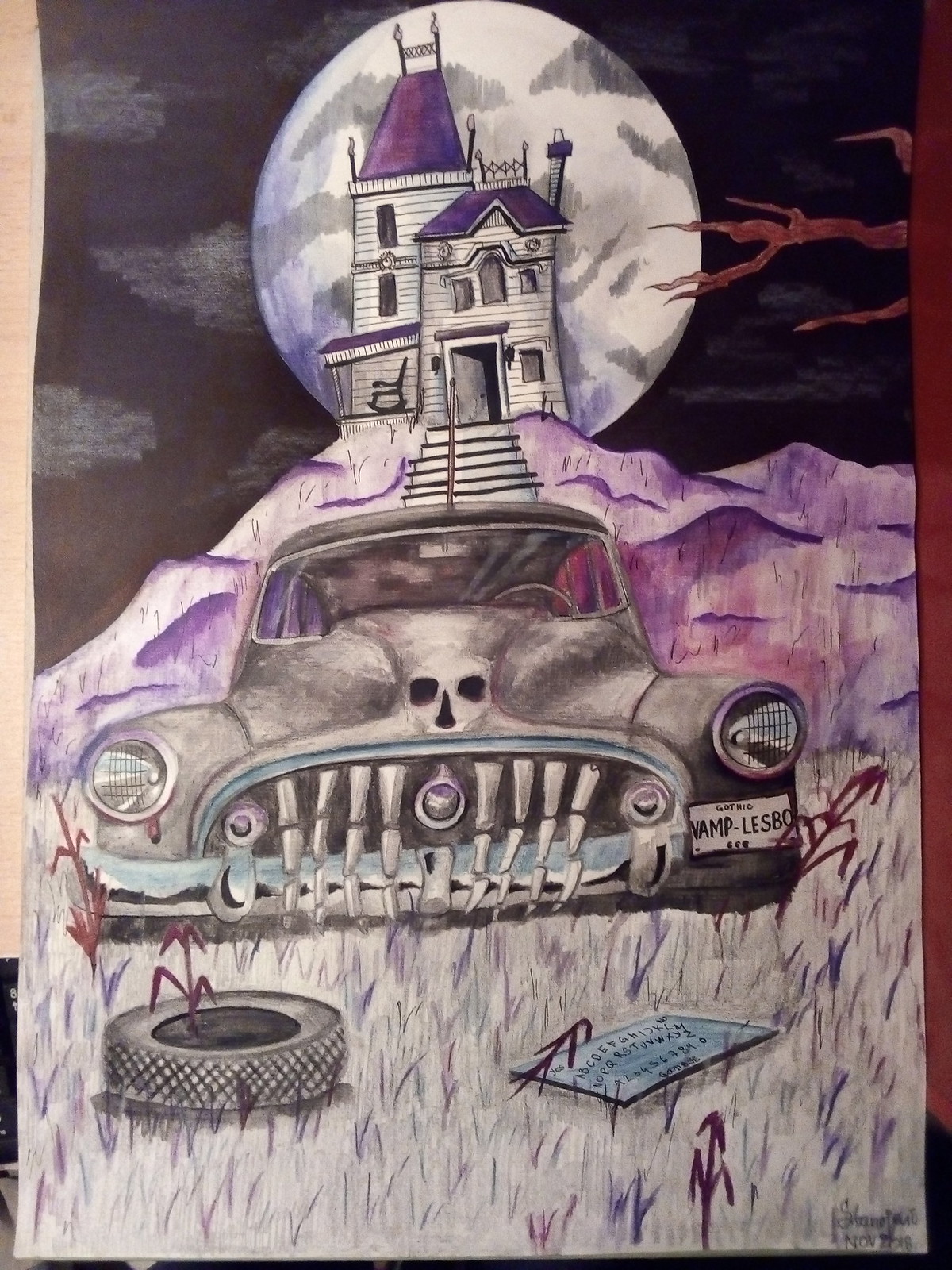This image captures a hand-drawn, cartoon-style scene centered on an eerie, haunted atmosphere. The crude drawing, with a washed-out signature dated November, is photographed on paper. Dominating the image is a 1940s to 1950s era car with an unsettling aesthetic: a skeleton head on the hood, a grill resembling metal teeth, and a license plate reading "GOTHIC VAMP LESBO." The foreground features a patch of grass in shades of white, purple, and blue, with an old tire overgrown by a purple plant and a blue piece of paper with writing. The background is encased in a sinister, almost black sky dotted with dark clouds and a luminescent moon casting eerie shadows. Perched on a purple hill stands a dilapidated mansion with a rocking chair on the front porch, a crooked roof, and twisted, wicked limb branches of an ominous tree. The overall scene evokes a strong sense of haunted desolation, blending elements of gothic horror with whimsical artistry.